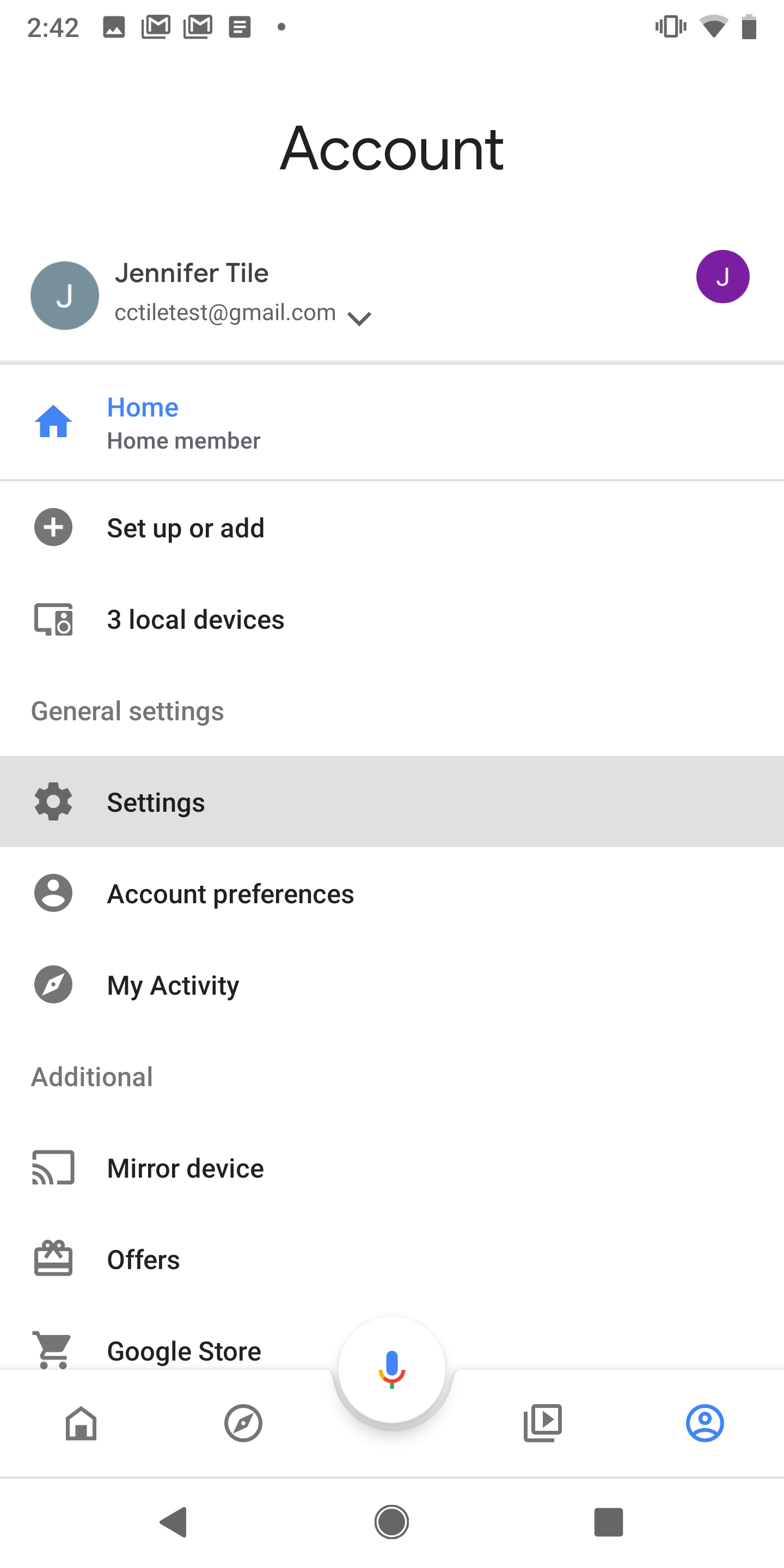This image depicts the account section of a smartphone screen, providing a comprehensive overview of the interface elements displayed. 

At the top of the screen, there's a timestamp showing "2:42" PM. To the right of the clock, several icons are arranged: a photos icon, two email icons, a pages/documents icon, a dot separator, followed by a triangle symbol, a vertical rectangle with three lines of varying lengths, a Wi-Fi icon, and a battery indicator.

In the middle part of the screen, the word "Account" is prominently displayed. Beneath it, there's a gray box containing a white letter "J". Adjacent to this is the name "Jennifer Tile" and the email address "cctiletiltest@gmail.com," followed by a dropdown arrow. Further to the right, there's a purple circle with a white letter "J" inside it.

Below this section, there's a blue home icon with the word "Home" next to it, and "Home Member" written underneath. A faint gray line separates this from the next section, which features an addition symbol labeled "Set up or add."

Next, an icon of a computer monitor and speaker is displayed with "Three Local Devices" listed to its right. Below that, in gray text, is "General Settings," and the settings icon has been highlighted. Following this, there's an "Account Preferences" section, next to which lies a user ID and a user photograph image.

Moving further down, there's an option labeled "My Activity," and beneath that, an "Additional Mirror Device" option paired with a Google Store link.

At the bottom of the screen, there is a navigation bar featuring several icons: a home icon, an unidentified icon, a microphone in the center, what appears to be a fast forward button, and another user profile icon. At the very bottom, there is a left-facing arrow, a home button, and a stop button for additional control functions.